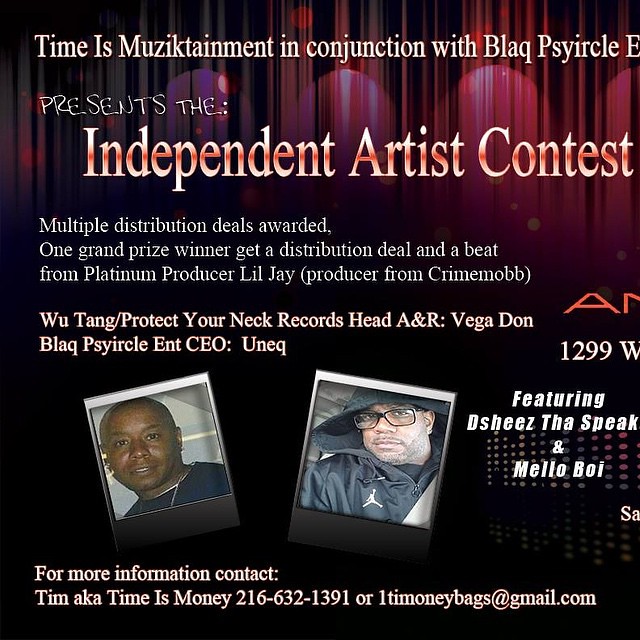This image is an advertisement presented by TimeIsMusic Entertainment in conjunction with Black Psyircle (B-L-A-Q-P-S-Y-I-R-C-L-E). The poster promotes an Independent Artist Contest, with a tagline that reads "Multiple distribution deals awarded." The grand prize includes a distribution deal and a beat from the platinum producer Lil' J, known for his work with Crime Mob. Notably, the contest is endorsed by Vega Dawn, the head A&R of Wu-Tang's Protect Your Neck Records, and CEO U-N-E-Q of Black Psyircle.

The background of the poster transitions from black at the bottom to reddish-purple curtains at the top. The text is predominantly white and gold, creating a striking contrast. Two photos are prominently featured at the lower part of the poster: on the left, a bald African-American man in a black shirt, and on the right, another African-American man with a short, well-trimmed beard, wearing sunglasses and a black Nike Jordan hoodie.

For more information, the poster provides contact details for Tim, aka TimeIsMoney, including a phone number (216-632-1391) and an email address (onetimemoneybags@gmail.com). The poster also features the names of D-Sheez, The Speak, and Mellow Boy.